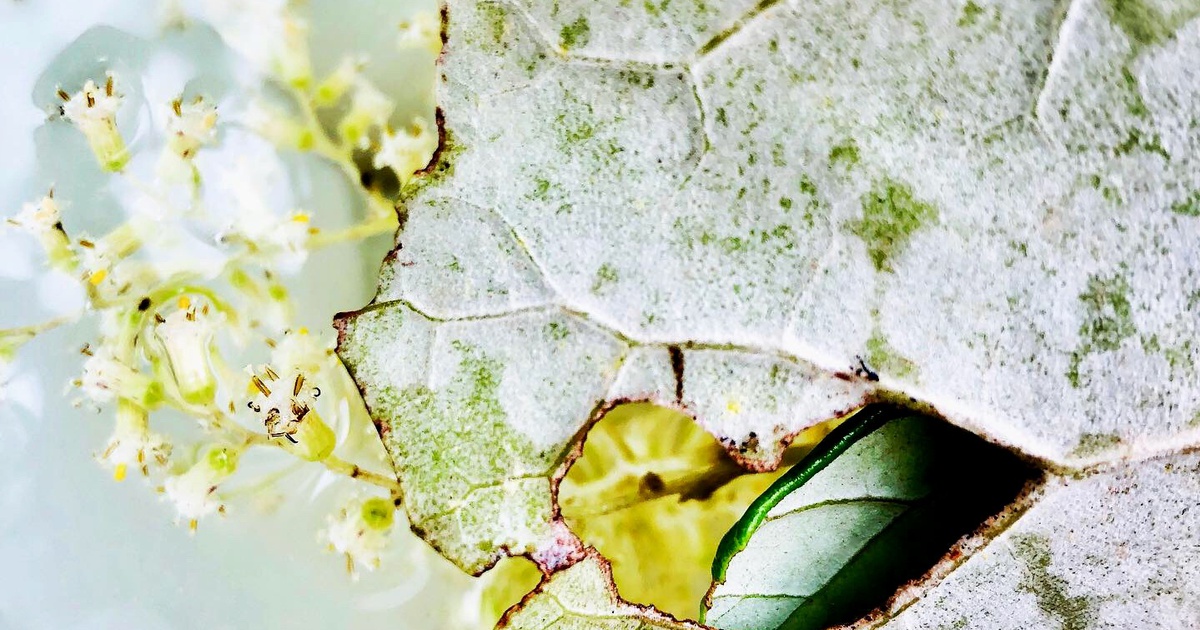The image, taken outside in the daytime, features a magnified or overly bright view of a plant on a white rock. On the left side, light green vines support delicate, white, bell-shaped flowers, reminiscent of honeysuckle, with tiny seeds protruding from their centers. To the right, a large leaf, marked by a striking contrast of green and white, appears wilted or affected by the lighting, revealing a dusty, white surface and green patches peeking through. Further down, a new leaf emerges, displaying a vibrant dark green hue. The rock beneath the plant shows green moss patches, adding to the natural texture. The background, a mix of pale bluish-green or gray tones, seems blurred with possible lens flare or glare, creating a soft, aquatic ambiance, suggesting proximity to water.